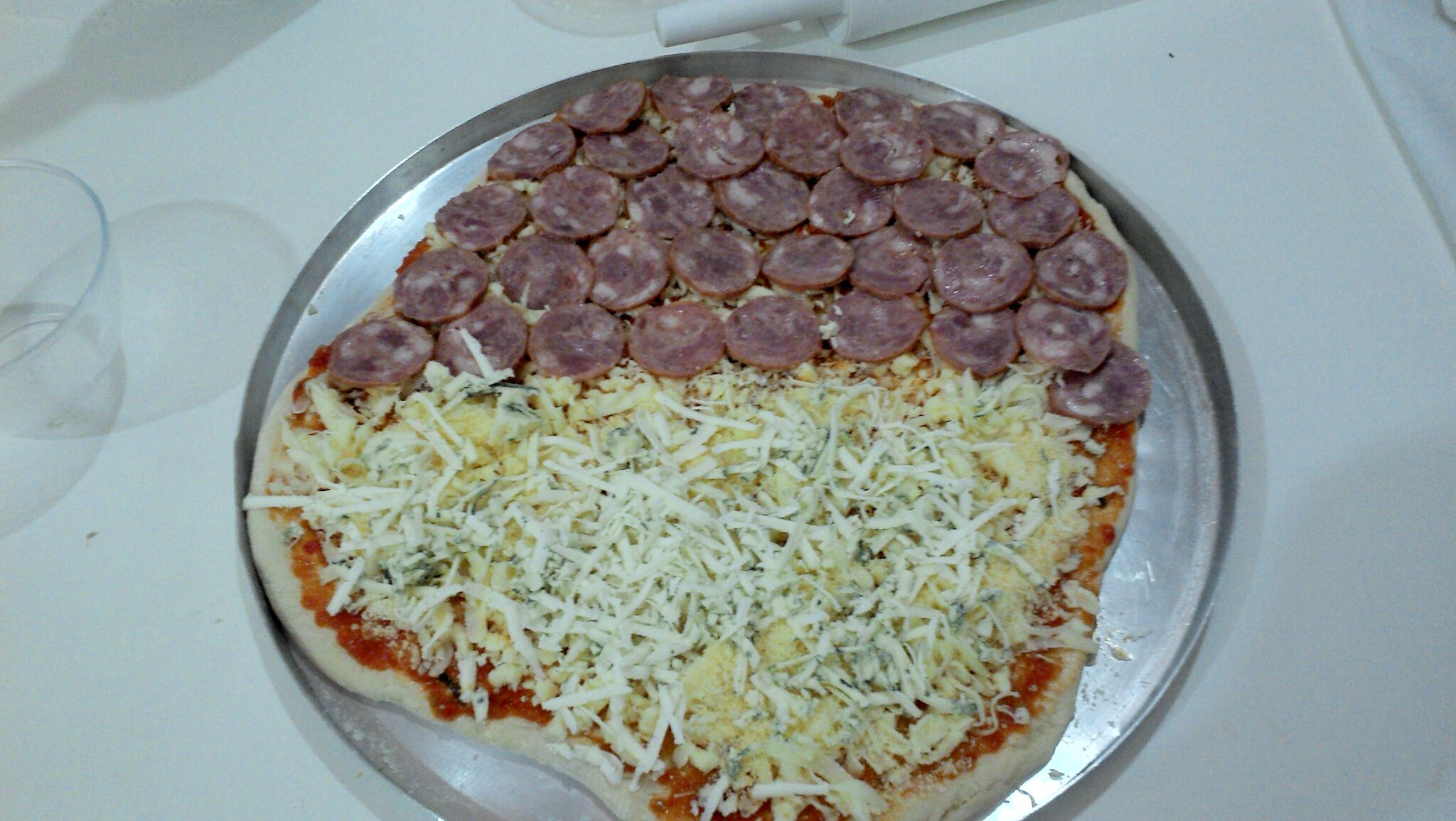The image depicts an uncooked pizza placed on a round silver baking tray. The dough, which isn't perfectly round, is topped with a rich marinara sauce and copious amounts of shredded mozzarella cheese, along with some other mixed cheeses. The top portion of the pizza is densely covered with small slices of pepperoni, nearly concealing the cheese beneath. The baking tray sits on a white surface, which might be a countertop or a table with a white tablecloth. To the left side of the image, there's a clear, empty glass, partially visible and casting a shadow onto the white surface.